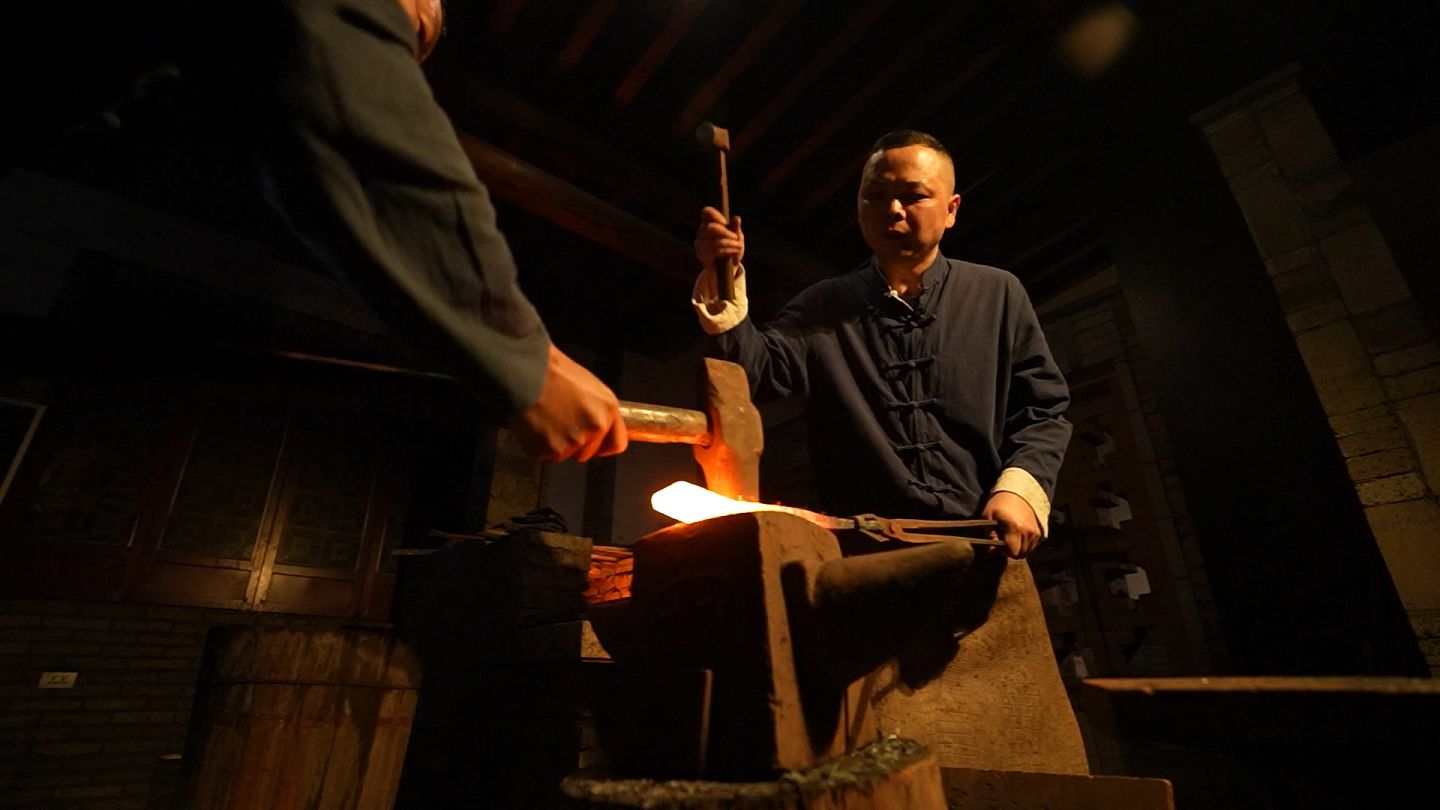The photograph captures two blacksmiths immersed in the meticulous craft of forging red-hot metal within a meticulously recreated historical setting. The backdrop features wooden panel shutters adorning the walls and robust brick pillars that add an authentic touch to the scene. 

The blacksmith directly facing the camera dons a brown leather apron over a mandarin-style navy blue jacket. With very short-cropped black hair, the Asian blacksmith is intently focused as he grips a hammer in his right hand while using calipers in his left to hold the glowing piece of metal resting on a sturdy base. 

To his right, only the arm of his companion is visible, wielding a larger, anvil-shaped hammer, also clad in a navy blue mandarin jacket. Together, they embody the timeless dedication and skill of blacksmiths, set against a rich tapestry of historical craftsmanship.